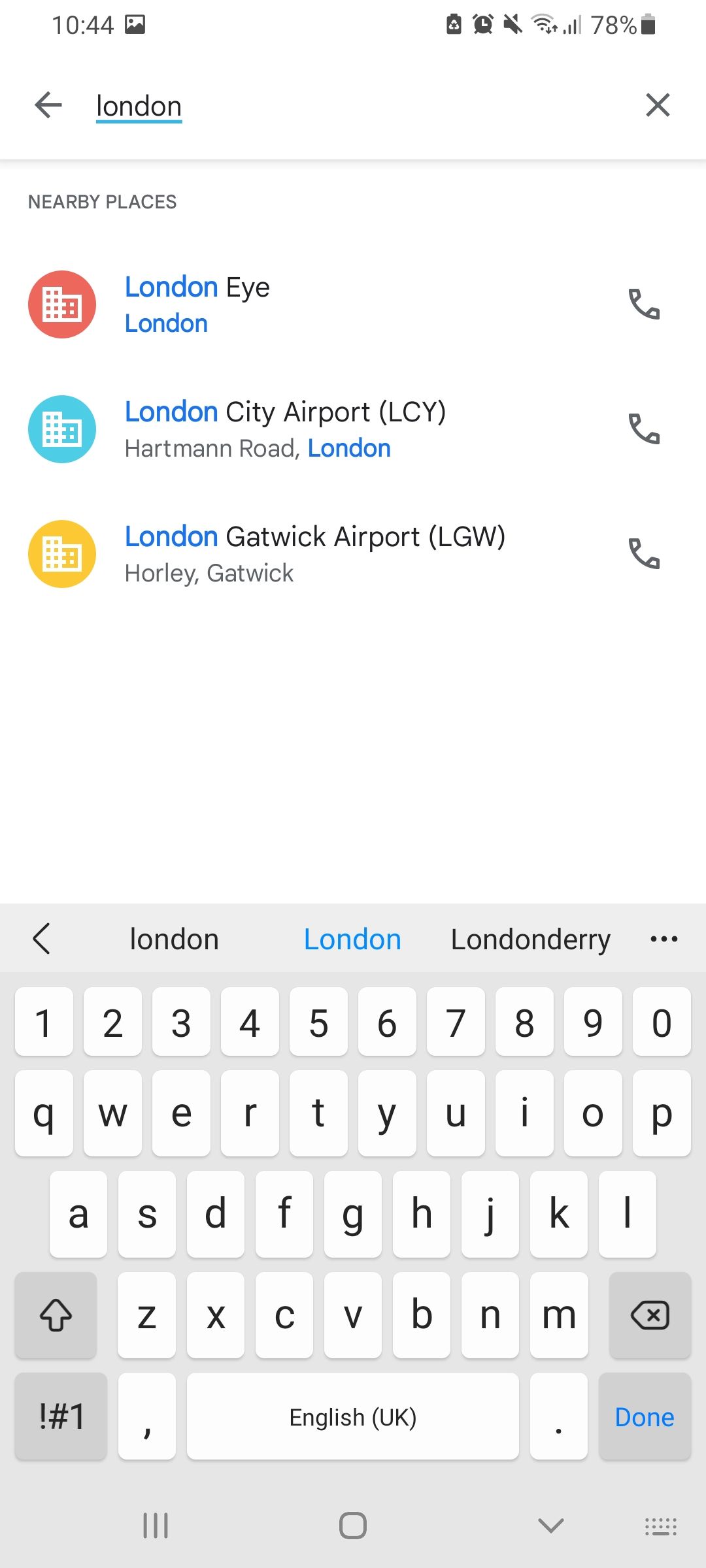This is a vertically oriented photograph, seemingly taken from a cell phone, as evidenced by the array of typical mobile interface icons. The background of the image is predominantly white. 

At the very top of the image, a horizontal bar displays several icons confirming the mobile source. Positioned on the top left is the current time, followed by an icon depicting a landscape. More centrally, there are several unfamiliar icons, but distinctly visible are an alarm clock, the Wi-Fi signal strength indicator, the cell phone signal strength bars, a battery icon, and a battery percentage indicator showing 78%.

Just below this, there appears to be a search query for "London," seen prominently with an arrow pointing to the left and an X on the right, enclosed within a gray-bordered box.

Further down is a section labeled "Nearby Places," accompanied by various icons and descriptions. The first entry is a red circle with buildings icon labeled "London", followed by a simple "I" and "London", with a phone symbol on the far right. The second entry features a turquoise circle with buildings icon, labeled "London City Airport," denoted by "L-C-Y" and further detailed with "Hartman Road, London" and a phone symbol on the right. The third entry is marked by a yellow circle with buildings icon, labeled "London Gatwick Airport," identified by "L-G-W" and specified as "Orleigh Gatwick," also accompanied by a phone symbol on the right.